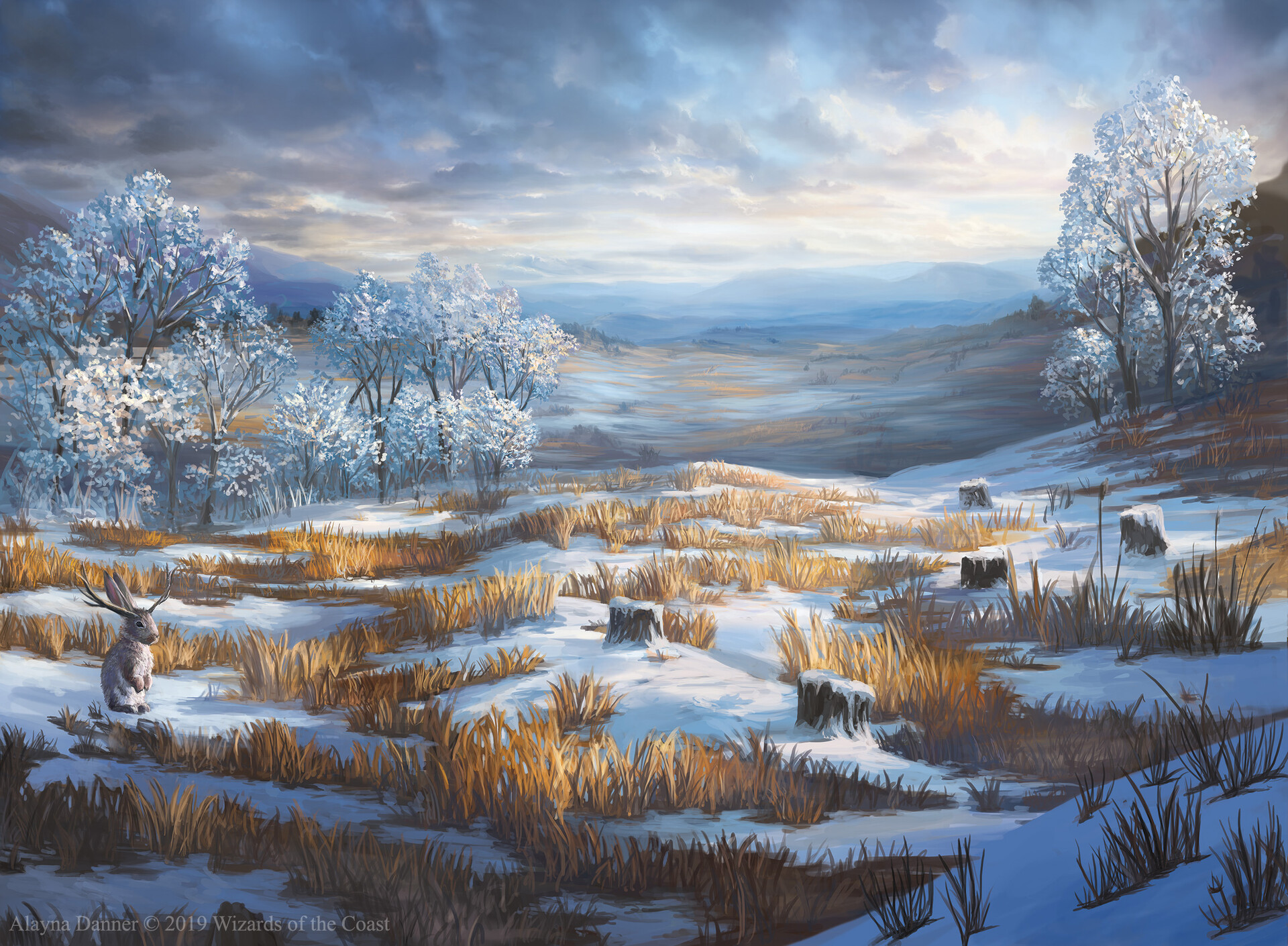This detailed, color illustration depicts a serene, snow-covered valley in winter. In the left foreground, a whimsical jackalope—a rabbit with antlers—sits amidst patches of snow, with tufts of yellow-brown grass poking through. Scattered tree stumps, also blanketed in snow, adorn the foreground. The mid-ground features a cluster of snow-covered trees stretching from the left to the right of the image, creating a natural frame. In the distance, subtle rolling hills and peaks rise under a sky tinged with blue and heavy with dramatic gray clouds. The wintry landscape, a prairie extending into a vast expanse, is rendered in a distinct artistic style, possibly painted or colored with pencils. The bottom left corner includes the text, "Alnia Donner, copyright 2019, Wizards of the Coast," signifying the illustrator and publisher.